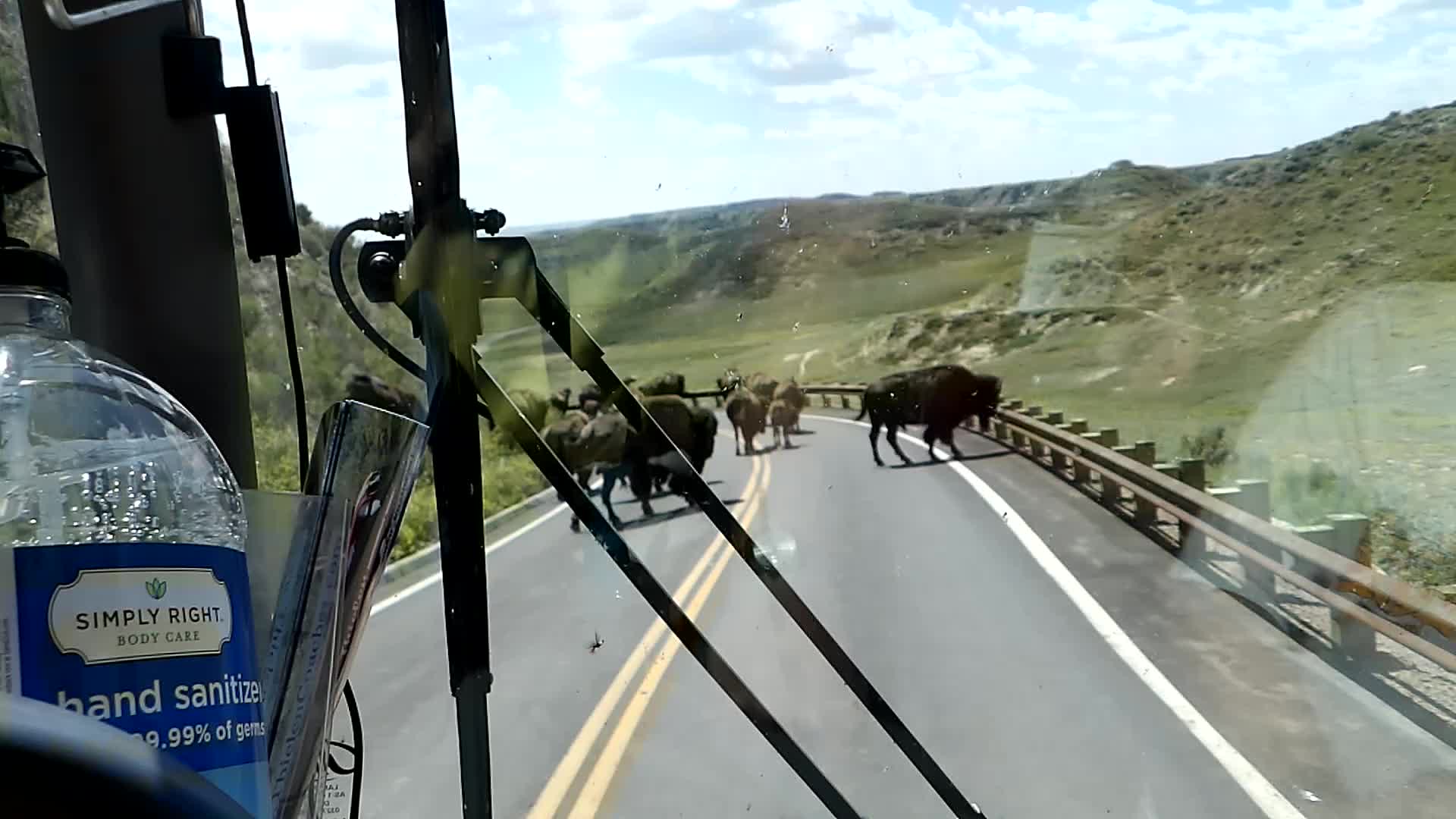The photograph captures a bright, sunny day on a two-lane mountain highway, surrounded by lush greenery and hills. The image is taken from inside a large vehicle, likely a bus or an RV, indicated by the presence of hand sanitizer near a gray vertical pole with black wires. The highway, marked with yellow center lines and white outer lines, is blocked by approximately a dozen bison in various shades of brown and black. These animals are scattered across the road, seemingly trying to cross despite a metal guardrail along the shoulder. The scenery outside the road shows a blue sky with scattered white clouds, and the terrain is a mix of grassy hills and rocky outcrops, adding to the picturesque yet interrupted journey.